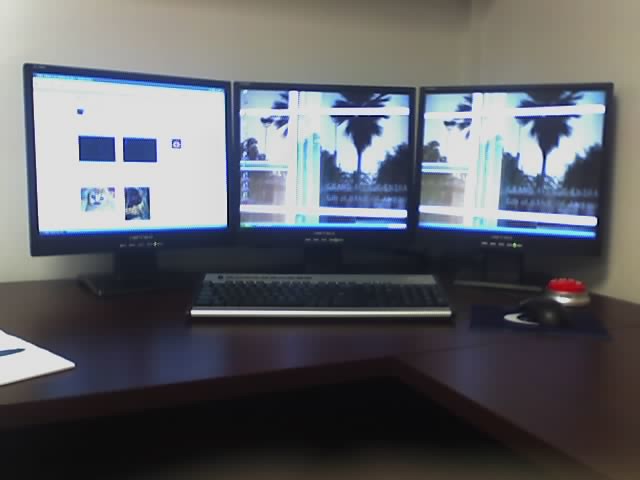The image depicts a dark brown, L-shaped desk positioned in the corner of a room with an off-white or light gray wall acting as a backdrop. Atop the desk sit three computer monitors arranged in a row, each with black frames and black rectangular pedestals. The center and right monitors display a tropical screensaver featuring palm trees and a wide blue body of water. The left monitor shows a web page with several open dialog boxes, possibly containing video thumbnails. In front of the center monitor is a silver and black keyboard, and to its right is a navy blue mouse pad with a white logo, complemented by a black plastic mouse with a red button. Scattered papers are visible on the left side of the desk, enhancing the lived-in workspace vibe. The photo is slightly blurry, but the vivid details of the desk setup are nonetheless discernible.